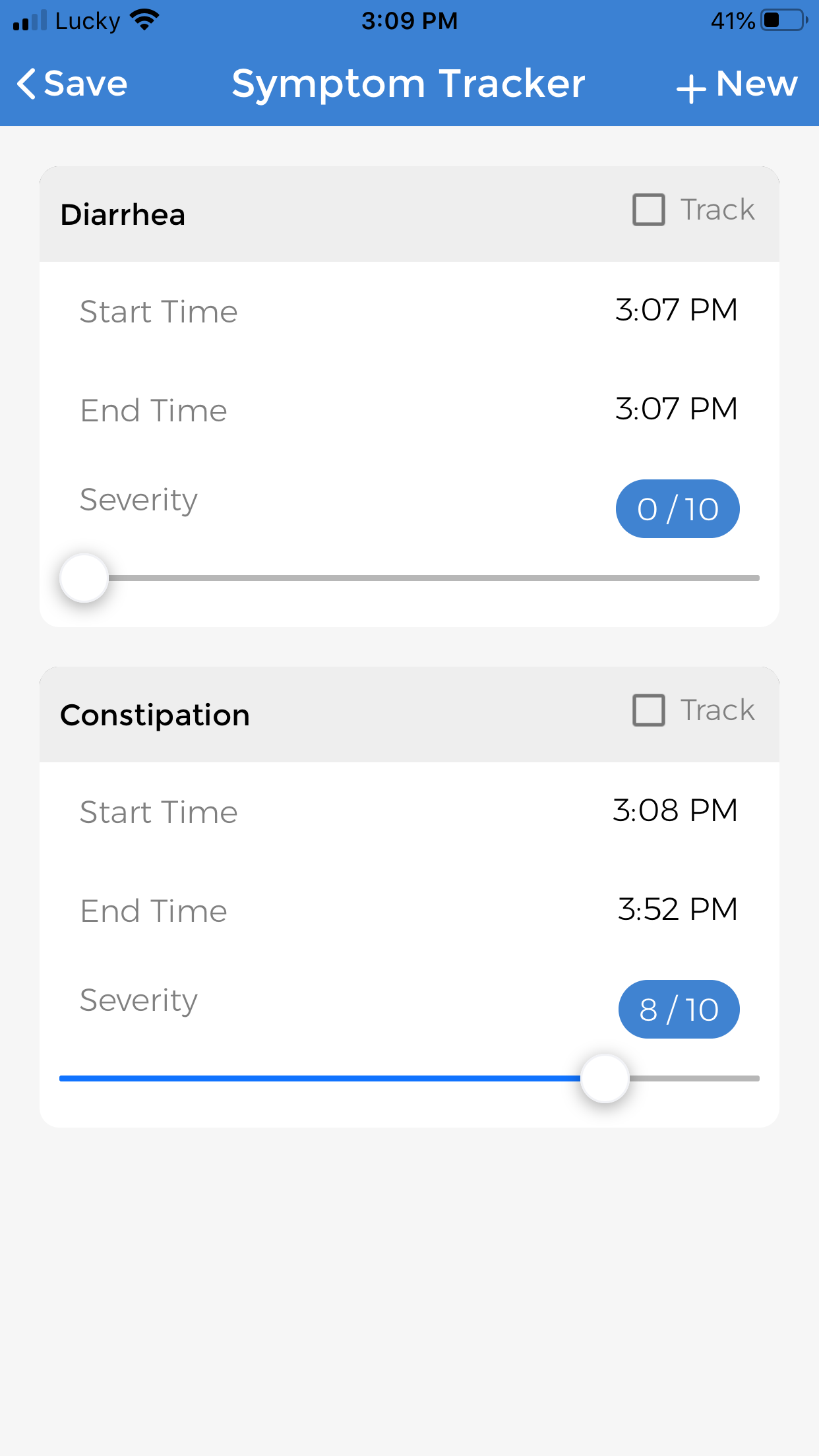This is a detailed screenshot from a mobile phone displaying a health application tracking symptoms. 

**Top Section:**
- The topmost blue bar features status icons and text information in black font. Starting on the left, it shows two out of five bars for Wi-Fi signal strength, followed by the word "Lucky," a full mobile signal icon, the current time of 3:09 p.m., and the battery level at 41%.

**Middle Section:**
- Directly below the blue bar, there is a header with navigation elements. On the left in white font, there is the word "Save" accompanied by a left-pointing arrow. Centered in the header is the title "Symptom Tracker." On the right side, there is a plus sign and the word "New."

**Main Screen:**
- The main part of the screen shows the application interface on a gray background. At the top, there is a darker gray triangle. Below this, in black font, the word "Diarrhea" is displayed with an adjacent clickable square box labeled "Track."
- Further down, information about the symptom is shown in gray font within a white rectangular box. It specifies:
  - Start Time: 3:07 p.m.
  - End Time: 3:07 p.m.
  - Severity: 0 out of 10, with an adjustable severity bar.
- Below the diarrhea entry, there is another symptom listed as "Constipation." The start time for this symptom is 3:08 p.m., and the end time is 3:52 p.m. (raising an interesting point about the duration and classification of constipation).

This detailed screenshot illustrates the functionality of the symptom tracking application, showcasing its user interface and the specific details it records for different symptoms.